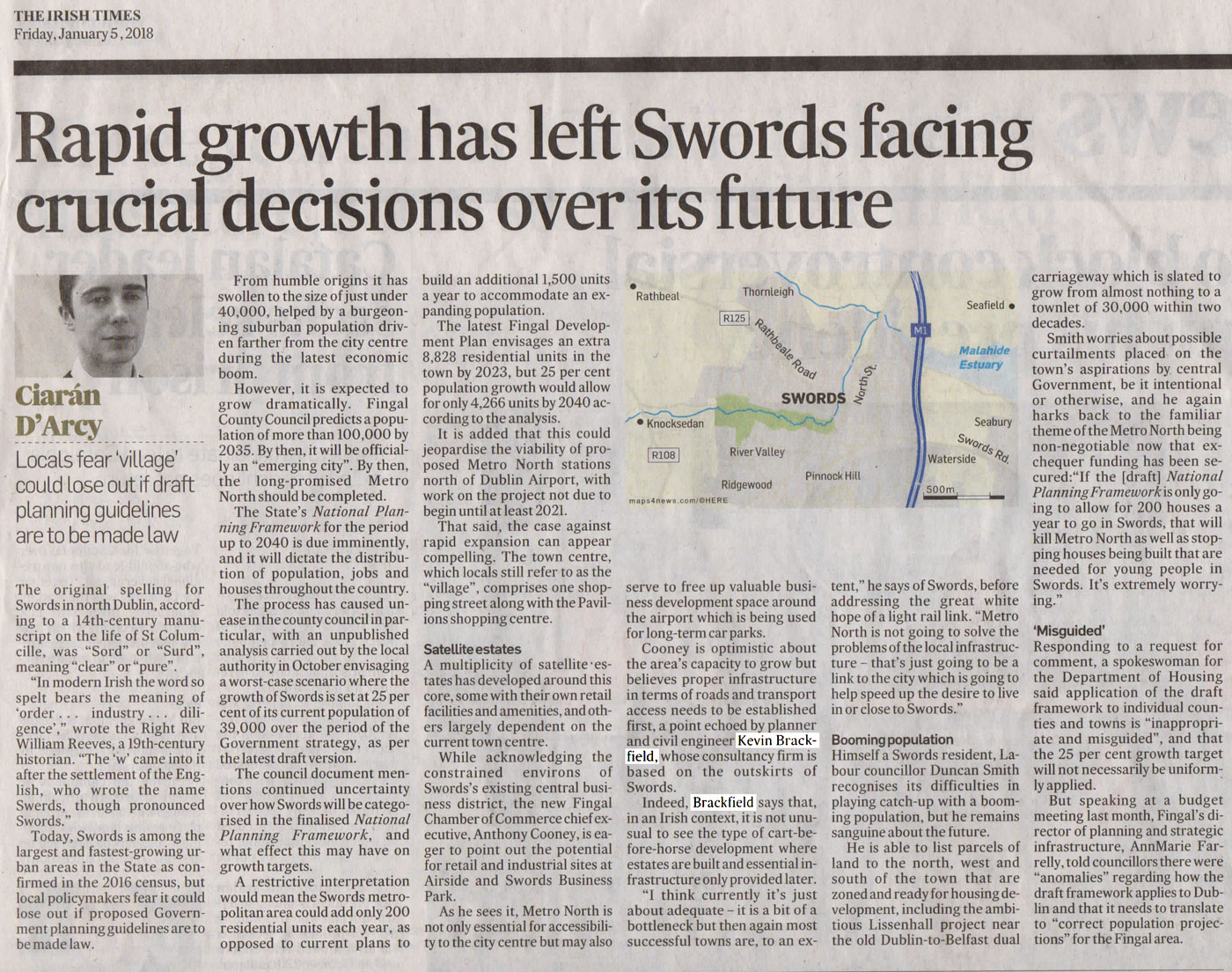This image features a newspaper article clipped from the Irish Times, dated Friday, January 5, 2018. The article, titled "Rapid Growth Has Left Swords Facing Crucial Decisions Over Its Future," discusses the challenges and concerns arising from rapid urban development in Swords, North Dublin. The article is detailed, featuring a photograph of a man identified as Claren DRC and mentions that locals fear the village could suffer if draft planning guidelines are enacted into laws. 

Highlighted within the text are mentions of Kevin Brackfield, emphasizing his role or quotes within the piece. Additionally, there is a map of Swords included towards the upper right of the article, showcasing various roadways, a lake or pond, and a waterway running through the area. The article mentions that the original spelling for Swords, according to a 14th-century manuscript of St. Clementsville, was "sword" or "surd" (S-U-R-D). The piece delves into historical context and current developmental pressures facing the community.